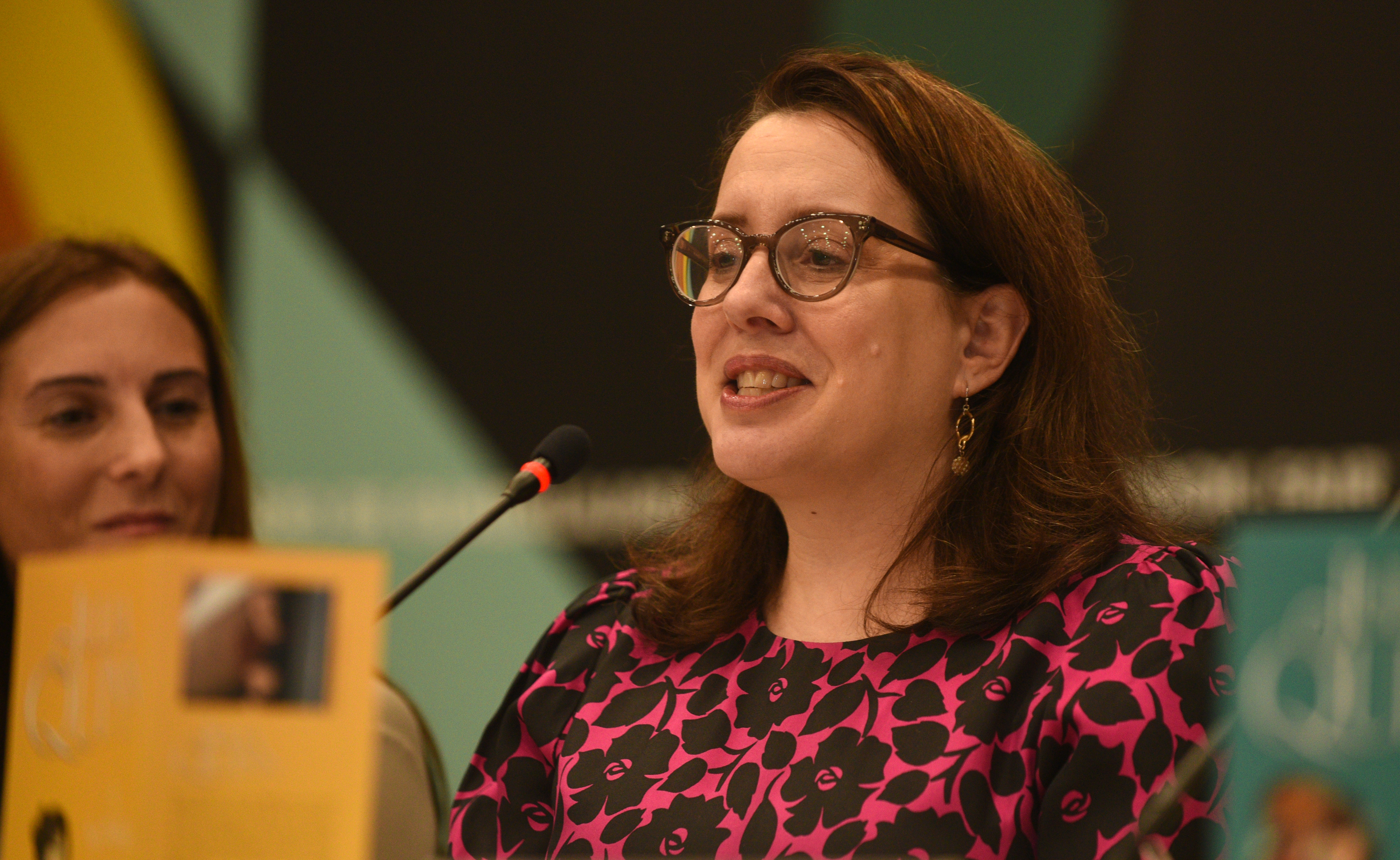In this photo, a woman with short brown hair and wearing eyeglasses is depicted at a podium, seemingly giving a speech. She is dressed in a pink and white blouse adorned with black floral prints. In front of her is a black and orange microphone and a blurred piece of paper, possibly with an image or a letter. To the left, another white female with brown hair and a big nose is smiling in her direction. Behind her to the lower right, a figure that appears to be a woman is adorned with an emerald green or turquoise wrap or scarf on her head. The background features a banner that is predominantly black in the middle with teal and yellow accents resembling diamond and circular patterns. The scene is indoors, as inferred from the lighting and setting, although it's not clear if it is daytime or nighttime.